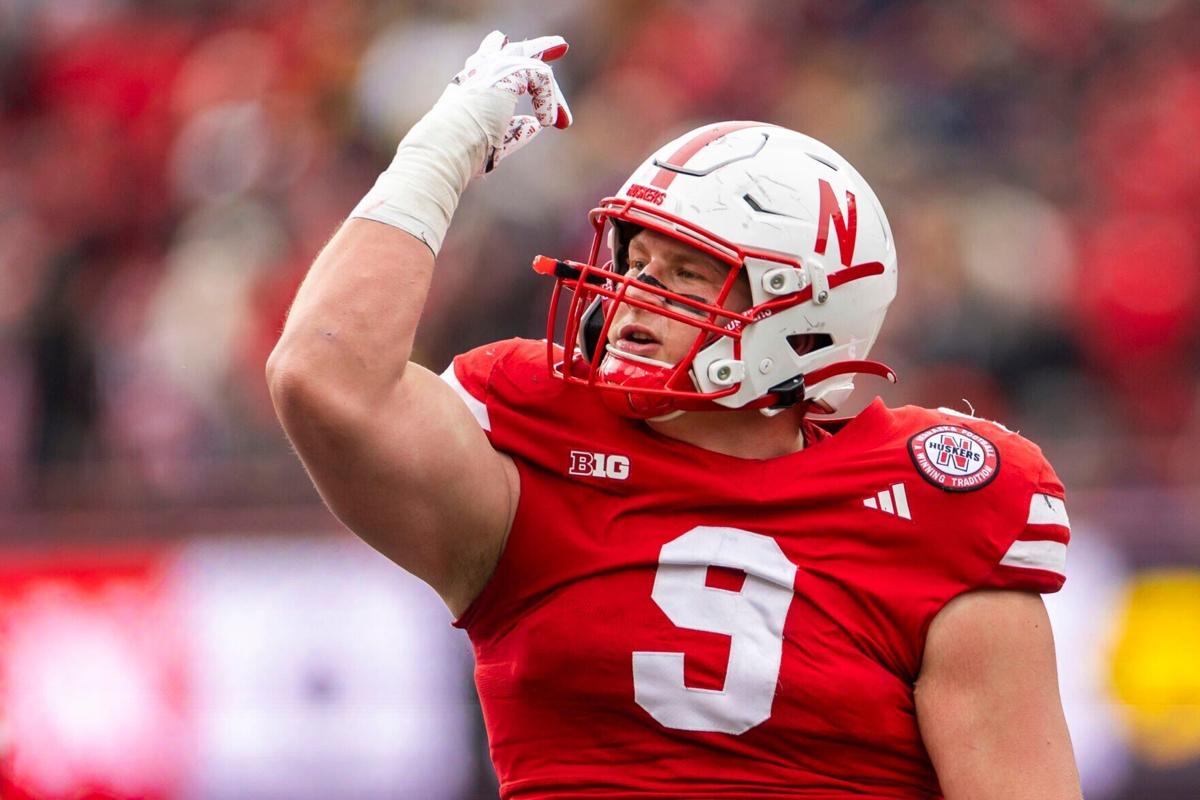In this up-close photograph of American football player Ty Robinson, he is captured from the ribcage up, wearing a red jersey with the white number nine prominently displayed at the center. His uniform includes a white helmet featuring a red mask and a red capital "N" on both the helmet and the jersey's patch, which reads "Huskers" alongside an Adidas logo. A "BIG" emblem is present on his right shoulder. Robinson's face is adorned with black paint across the bridge of his nose and under his eyes, enhancing his intense focus. His body faces the viewer while his head is turned to the right. He is energetically lifting his right arm, bent at the elbow with a wrapped wrist and a gloved hand. His left arm hangs at his side. The blurred background, a mix of reds, whites, browns, and yellows, suggests the presence of the crowd and stadium billboards, evoking the vibrant atmosphere of a Nebraska football game.